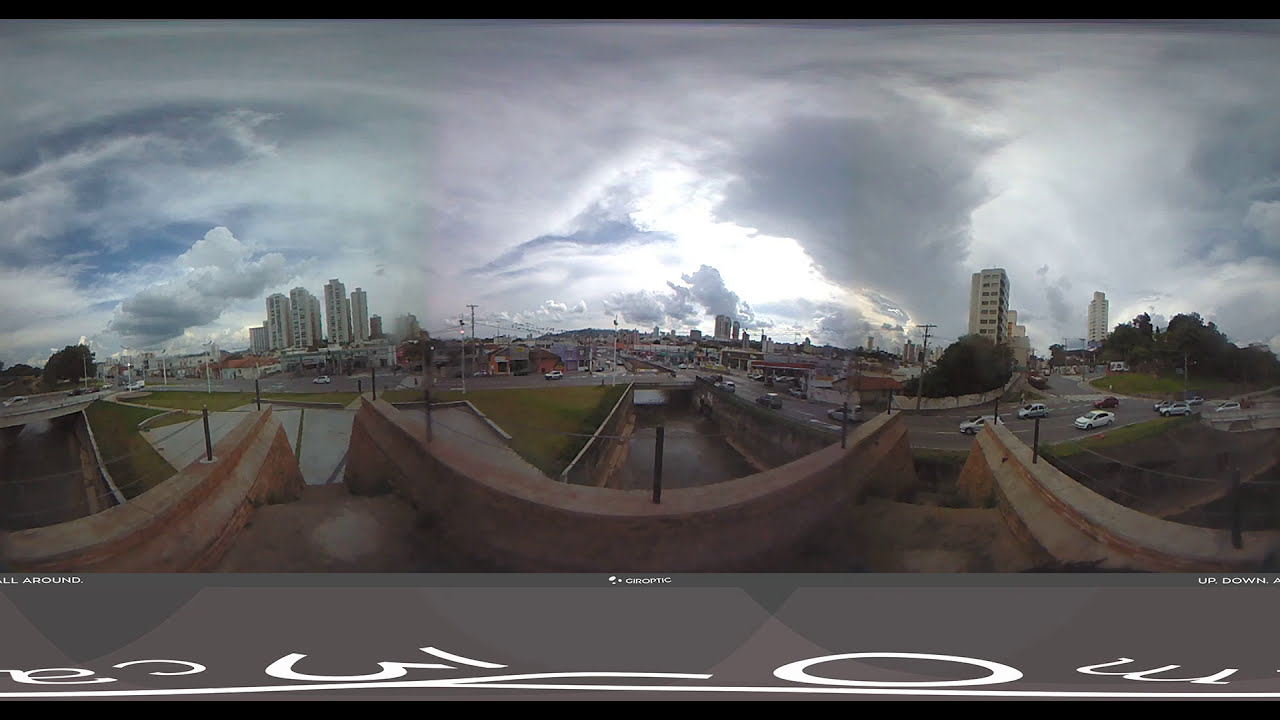The photograph, likely taken with a slightly distorted webcam from an outdoor vantage point, captures a panoramic view of a bustling city during a cloudy day. The image is vertically oriented and bordered by thin black lines at the top and bottom, with a wide gray strip featuring indistinct white lettering at the bottom. Dominated by an overcast sky, the clouds range from gray to white and appear heavy with impending rain, tinged with shafts of light piercing through in some areas.

In the foreground, there is a low concrete wall with curved features and narrow concrete stairs descending alongside some railings. This indicates the nearby structure where the camera might be mounted. Extending into the middle ground, the city streets teeming with traffic, including around 10 to 20 cars, intersect the scene. Diverse buildings fill the background: on the left side, there's a cluster of large white skyscrapers with numerous windows, transitioning to smaller buildings towards the center, and finally two more prominent white skyscrapers on the right. Sprinkled throughout the cityscape are green trees, enhancing the urban environment's freshness. The leftmost and rightmost sections of the image also show more tall buildings further in the distance, contributing to the dense urban skyline.